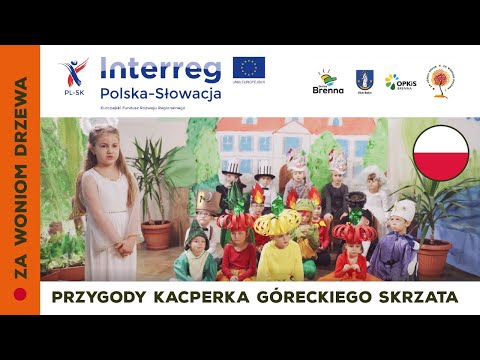The image depicts a landscape-oriented advertisement with a thick black border at the top and bottom. Centered at the top on a white background are the blue letters "INTERREG," followed by "POLSKA STOWARZYSZENIE" written underneath. To the right of this text are several logos, including a blue shield and the names "BRENNA" and "OPKISS." The top section also features a blue flag adorned with a circle of yellow stars.

A prominent orange vertical stripe runs along the left side of the image, containing text in another language, likely reading "ZA WONIOM DRZEWA." Below the top white border, the central part of the image shows a young girl with long blonde hair standing on the left, wearing a white dress with her hands clasped at thigh level. Positioned in front of a classroom setting, she faces a group of seated children who are dressed in vibrant costumes resembling fruits, vegetables, and even some in top hats. The costumes include colors such as green, red, yellow, and purple. Additionally, there are potted plants placed between the girl and the group as well as on the far right side of the image. At the bottom, above the black border, more text is displayed on a white background.